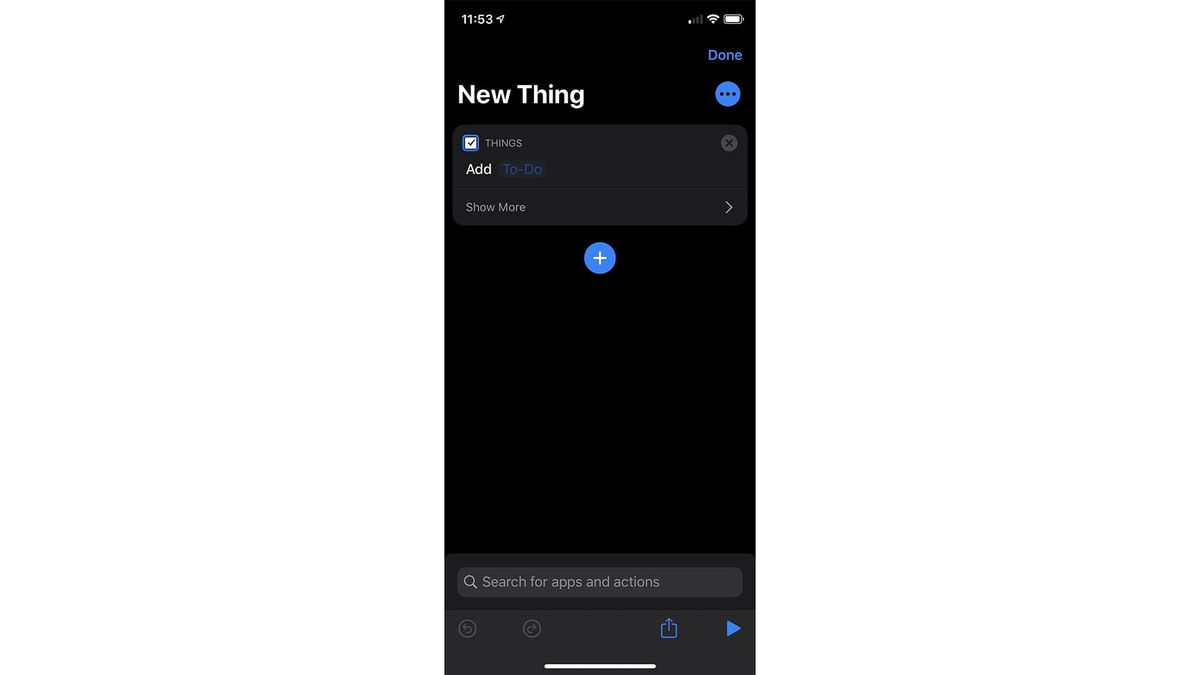The image is a screenshot of a smartphone interface, captured in night mode, with a predominantly black background. In the top left corner, the current time is displayed in white, while on the right, a status bar shows one cellular signal bar, a strong Wi-Fi signal, and a mostly charged battery icon. Just below these icons, there is a blue "Done" button on the right side of the screen. To the left, bold white letters spell out "New Thing," accompanied by a vertical three-dot menu icon within a blue circle.

Beneath this title, the word “Things” appears in gray, next to an “X” icon, suggesting it's a list management app. A prompt to “Add To Do” is present, followed by a "Show More" option with a right-facing arrow. Below this, in the lower third of the screen, a white plus sign inside a blue circle offers an additional way to add items.

Further down, a gray search bar rectangle appears, slightly lighter than the background gray. The search bar contains a white magnifying glass icon on the left, with the placeholder text "Search for apps and actions" in a light gray or white font. Underneath, the menu in a darker gray section displays a blue arrow pointing to the right and a blue square with an upward left-pointing arrow. At the very bottom, the phone’s menu button is visible, depicted as a white vertical line. Two other unidentified icons, also in light gray, are positioned to the left side of this line.